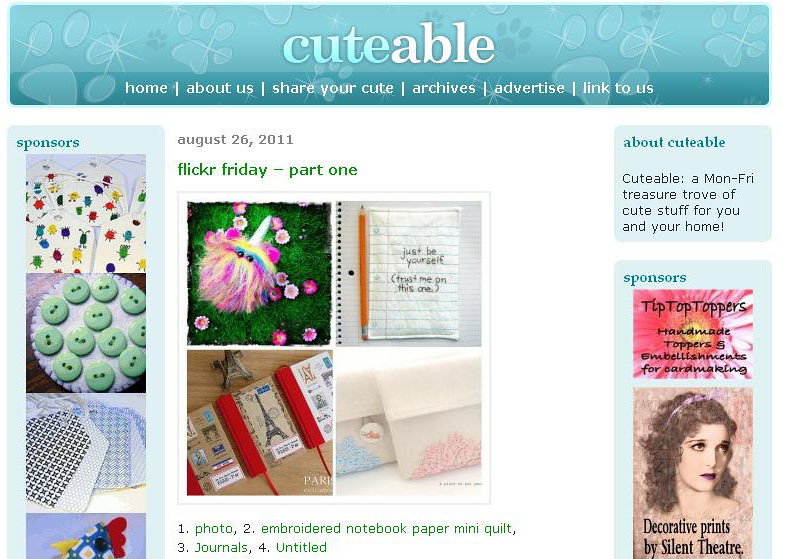The image captures a screenshot from a website called "Cutable," characterized by a simple design. At the top, a blue rectangular box adorned with paw prints displays the site’s name prominently, where "Cute" is written in blue and "able" in white. Below the title is a white menu bar featuring options like Home, About Us, Share Your Qt, Archive, Advertise, and Link to Us. The main section of the webpage, dated August 26, 2011, highlights a blog entry titled "Flickr Friday Part 1." This section includes a mosaic of four pictures showcasing various customized items including furry toys and lookbook pages.

On the left side, a column titled "Sponsors" features three images: the first displays colorful insect drawings, the second shows a white circular shape adorned with numerous light green buttons, and the third presents layered patterns resembling stacked paper sheets. The right column mirrors the left, displaying a series of sponsor images that include various decorative and customizable items such as buttons, embroidered notebook paper, and stationery. The entire page is set against a clean white background, providing a clear and organized look at the diverse offerings and featured content.